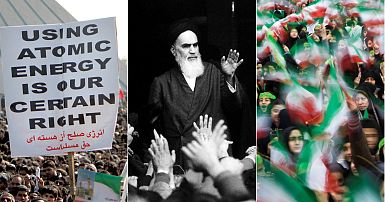This composite image is divided into three equal sections, showcasing significant moments in Iran, likely during its revolution. The left section is a color photograph capturing a protest scene where a large crowd can be seen behind a prominent white sign with black text reading "Using atomic energy is our certain right," accompanied by red Islamic script underneath. A sloped gray surface, possibly a roof, is visible in the background. The middle photograph is in black and white and depicts Ayatollah Khomeini in his black robe and white beard, waving to a crowd that responds with raised hands. The right section returns to color and displays another protest dominated by women in black head coverings, waving Iranian flags that feature green, white, and red stripes. The atmosphere in this part appears patriotic, signifying a strong sense of nationalistic fervor.